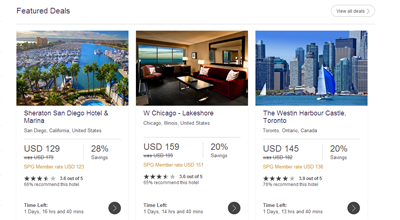The image is a screen capture from a travel or hotel booking website, featuring a "Featured Deals" section showcased on a clean white background. In the top left corner, blurred gray lettering displays the title "Featured Deals," and in the upper right corner, an oval gray button is outlined with the text "View All Deals."

Below this header are three horizontally aligned images, each representing different travel deals.

1. The first image on the left is an aerial view of a municipal cityscape surrounded by water, slightly blurry, with a visible swimming pool in the bottom right corner. The caption below this image reads "Sheraton San Diego Hotel and Marina" in black text. This deal offers a stay at the Sheraton for USD $129, which includes a 28% savings. It is rated 3.5 stars.

2. The central image portrays an interior space resembling a high-end office or an office waiting room, primarily decorated in shades of brown and black. The accompanying text states "W Chicago Lakeshore," where rooms are available at USD $159, reflecting a 20% savings. This hotel also has a rating of 3.5 stars.

3. The final image on the right is captured from a waterway perspective, showing skyscrapers along the shoreline of a major city. The caption indicates "The Westin Harbor Castle, Toronto," with a rate of USD $145 and a 20% savings. This option enjoys a 3.9-star rating.

Below each listing, to the right, is a dark gray circle featuring a white right-facing arrow indicating the time left for the deal.